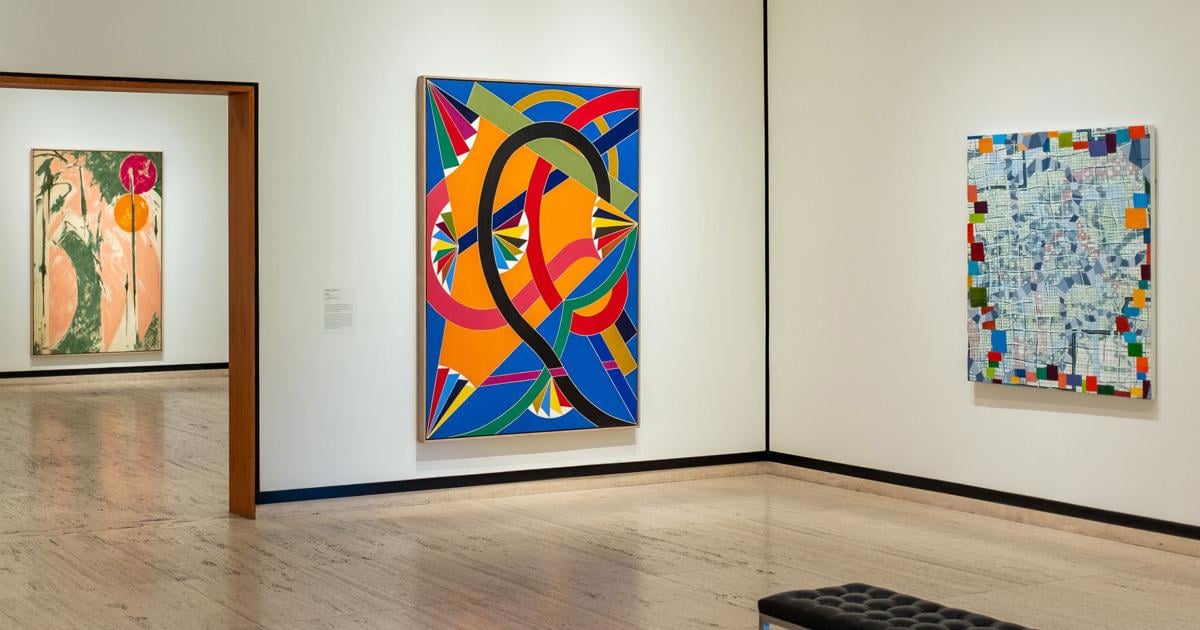The photograph captures the interior of an art gallery featuring two connecting rooms. The gallery has light blonde, pale brown wooden floors and dark white walls with brown trim. In the foreground, part of a black, padded bench for seating, typically found in art galleries, is visible.

In the main room, three large paintings adorn the walls. On the left, there is a vivid modern art piece with a blue background showcasing various colorful geometric shapes in yellow, green, red, pink, purple-pink, dark blue, and pale green. Toward the center, a similar abstract piece employs bold colors and shapes, prominently featuring bright blues, reds, and greens, akin to a hand-drawn city map with a complex interplay of geometric forms.

On the right, another painting with a blue background is adorned with several small lighter blue, black, green, and orange tiles, arranged around its perimeter. Through a hallway in the background, a painting with cream and green-colored swirls, along with a grey line featuring a yellow and pinkish ball, is visible. This artwork displays subtler tones in shapes suggesting a peach-colored human form with a reddish-pink head and an orange blob, adding to the abstract nature of the exhibition. The overall spaciousness and careful arrangement of art pieces provide an immersive experience for gallery visitors.